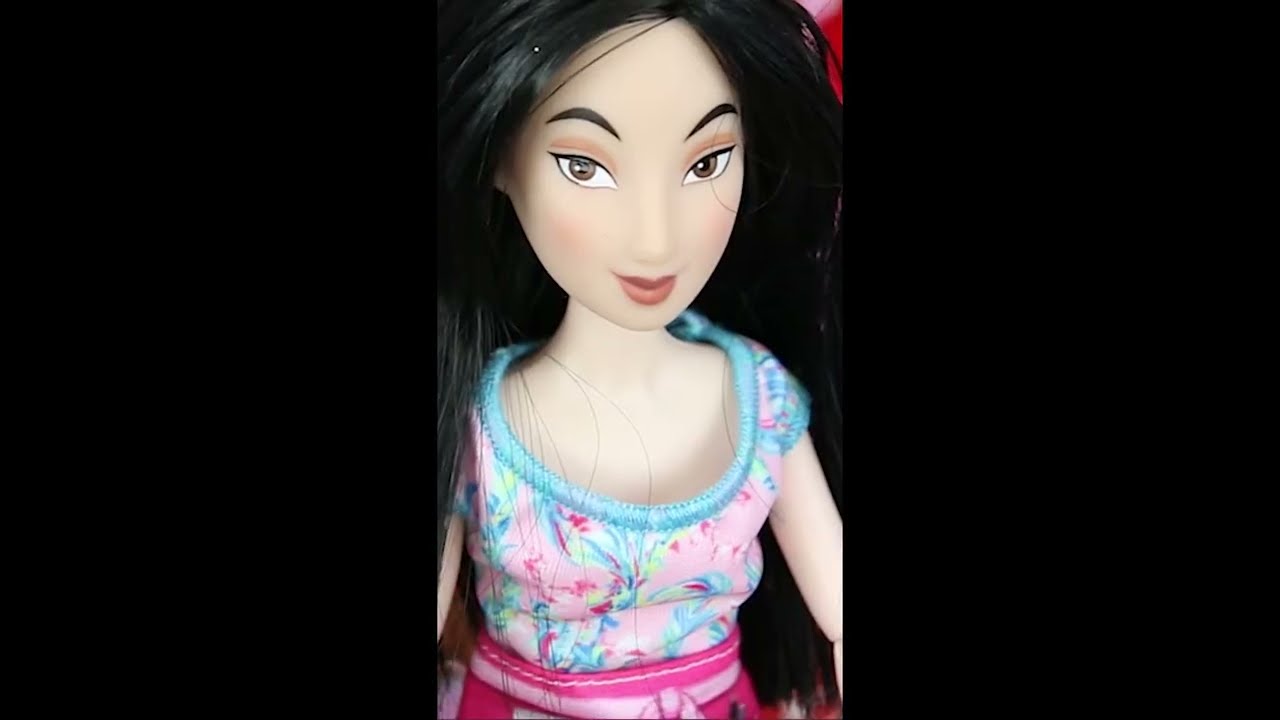The image features a close-up portrait of a doll that resembles Disney's Mulan, showcasing an Asian or Middle Eastern aesthetic. The doll has long, straight black hair, and distinctive brown eyes that are slightly slanted, with black, high-arched eyebrows. Her lips are pink and closed in a serene expression. She wears a short-sleeve shirt with a large round neckline, adorned in a pink and blue floral pattern, and below that, she sports pink pants or a skirt. The background is solid black on both sides, which frames the doll centrally and emphasizes her features and attire. Only the upper half of the doll, from the waist up, is visible in this photograph.